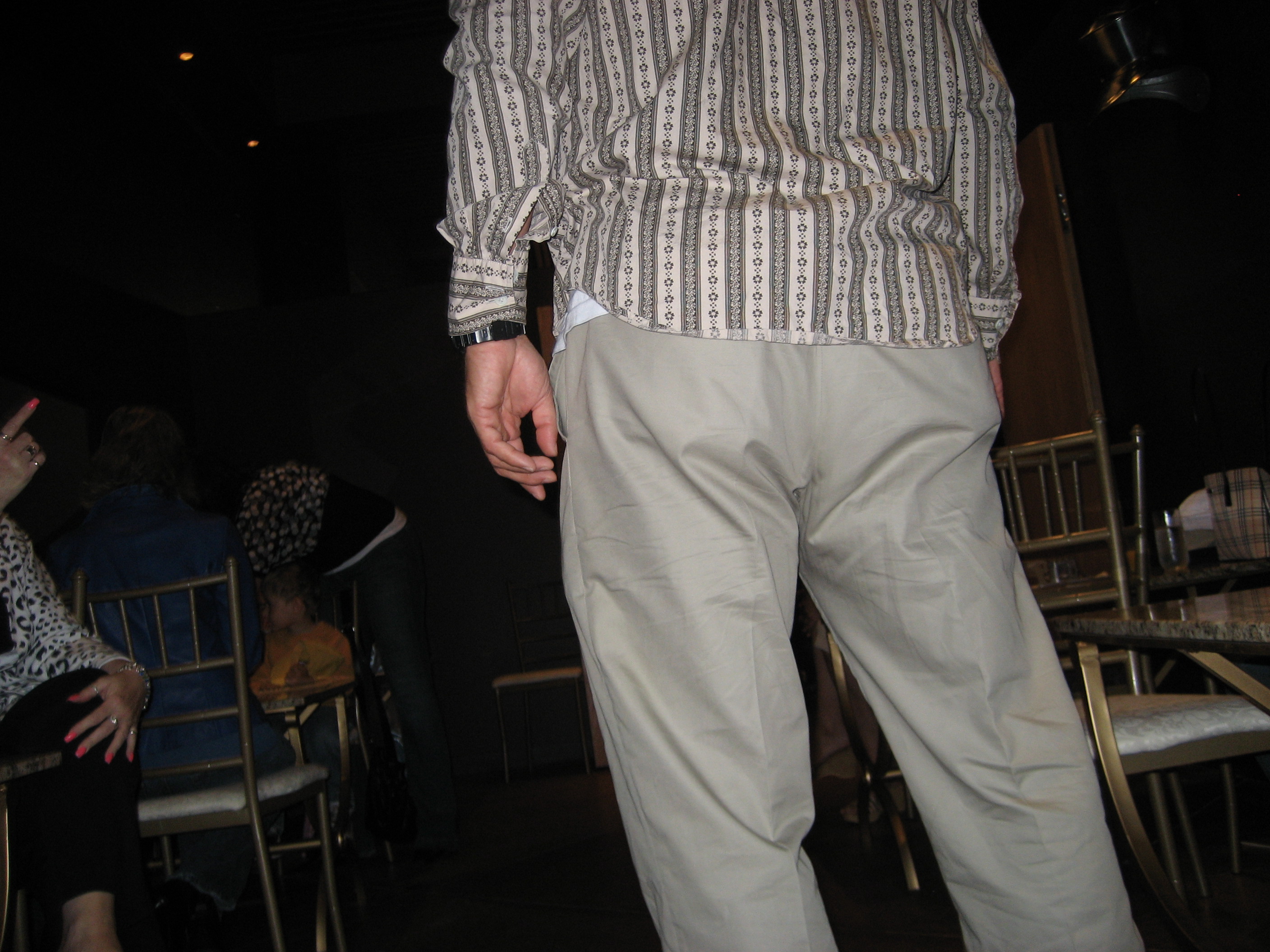This indoor photograph captures a dimly-lit, social setting at night, centered around an individual standing with his back to the camera. The man is dressed in a vertically striped button-up shirt, featuring cream and olive green hues, paired with beige khaki pants. His left wrist sports a black watch, and his hands rest at his waist. Surrounding him, both to the left and right, are thin metal chairs with white padding arranged around round tables. On the far left, a woman's hands are visible; she has hot pink nail polish, wears several rings and bracelets, and points towards the man. She is partially seen with black pants and an animal print black and white blouse. The background is predominantly dark and shadowy, highlighted by minimal track lighting on the ceiling. Additional figures can be seen in the shadowy depths, including a child in a yellow shirt and another person in a blue jean jacket, blending into the dark ambiance.